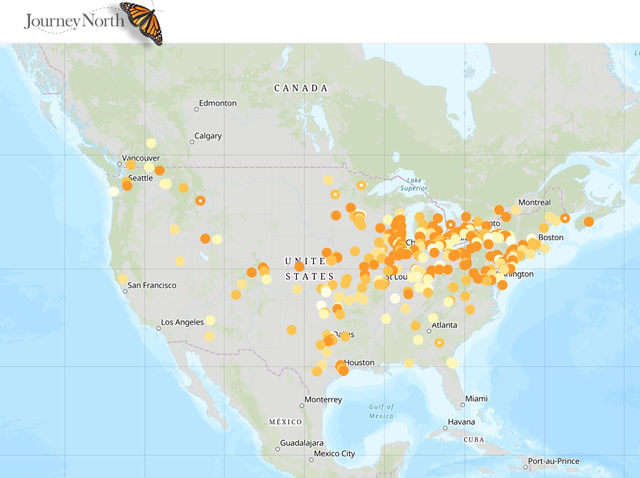This is a digitally created map image depicting North America's geography with a focus on butterfly migration routes. The map primarily showcases Canada, the United States, and Mexico, with land masses rendered in varying shades of brown and water bodies in light blue with subtle white outlines. The background features a grid pattern made up of square shapes separated by thin gray lines.

At the top of the map, "CANADA" is inscribed in small black letters, with significant cities like Edmonton, Calgary, and Vancouver marked with circles. Moving south, cities such as Seattle, San Francisco, Los Angeles, Monterrey, Guadalajara, Mexico City, and numerous others like Havana, Port-au-Prince, Miami, Atlanta, Washington, Boston, Montreal, Toronto, and St. Louis are labeled.

The map is sprinkled with numerous small, differently colored circles—ranging from beige, tan, light green, orange, dark orange, to light yellow—indicating various points of interest. These dots are notably denser in the Midwest and Northeast regions, suggesting a cluster of activity or migration routes. Additionally, a butterfly is depicted in the top left corner of the map, emphasizing the theme of the monarch butterfly's journey northward. The overall style and distribution of dots suggest it is illustrating the concentration and pathways of the butterfly migration.